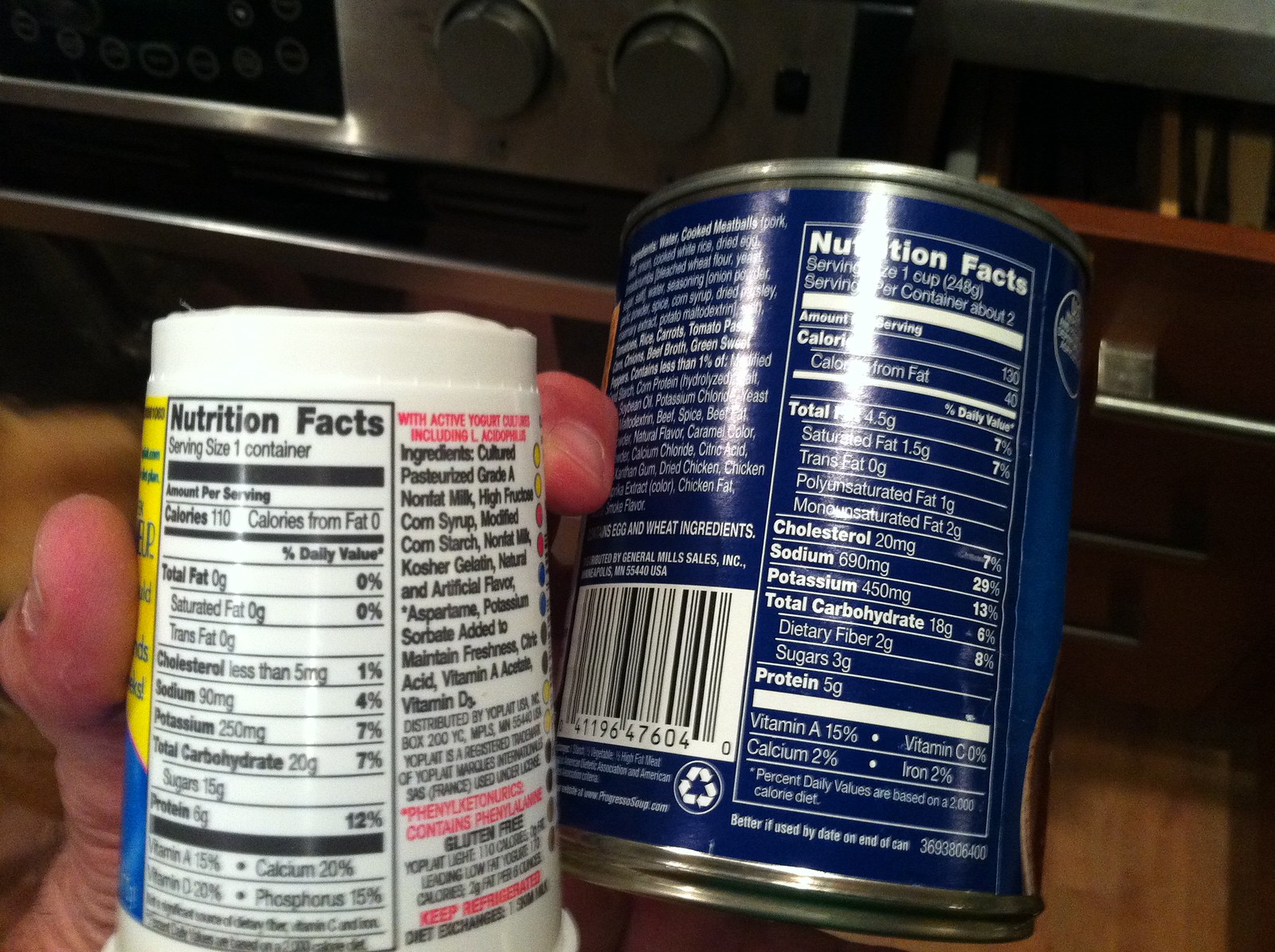In this close-up, rectangular photograph, we observe a Caucasian hand with short nails gripping a white container of yogurt. The thumb and pointer finger are clearly visible as they securely hold the container. The label on the yogurt container is readable and displays detailed nutritional facts: serving size 1 container, 110 calories, 0 calories from fat, 92 milligrams of sodium, less than 5 milligrams of cholesterol, 15 grams of sugars, and 6 grams of protein. It also mentions the presence of active yogurt cultures, including acidophilus, and lists ingredients such as cultured, pasteurized, grade A nonfat milk, high fructose corn syrup, and modified corn starch.

To the right of the yogurt container, partially visible, is a blue can. The specific food type on the can is unclear, but the nutritional information notes 130 calories per serving with 2 servings in the container. Additional details include 690 milligrams of sodium and 450 milligrams of potassium. A portion of the label, in the lower left corner, reveals the General Mills logo and lists some ingredients, including egg and wheat.